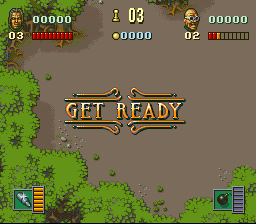This digital image captures the opening screen of a video game. Dominating the left and right sides of the screen are numerical scores represented by five zeros, placeholders for where the players' points will accumulate. Below this score line runs a bar, setting the stage for the upcoming interaction. 

To the left of the bar is an image of contender number three, identified by the numeral "03" displayed prominently at the top. This contender has long hair cascading smoothly. To the right, contender number two is showcased. This contender sports glasses and embodies a rather eccentric appearance. 

At the center of the screen, a large "03" stands out, possibly indicating an initial score or round number. Below, in bold yellow and orange text, the command "Get Ready" grabs attention, signaling the imminent start of the game. Borders of lush simulated greenery wrap around the edges of the screen, immersing the viewer into an engaging virtual environment.